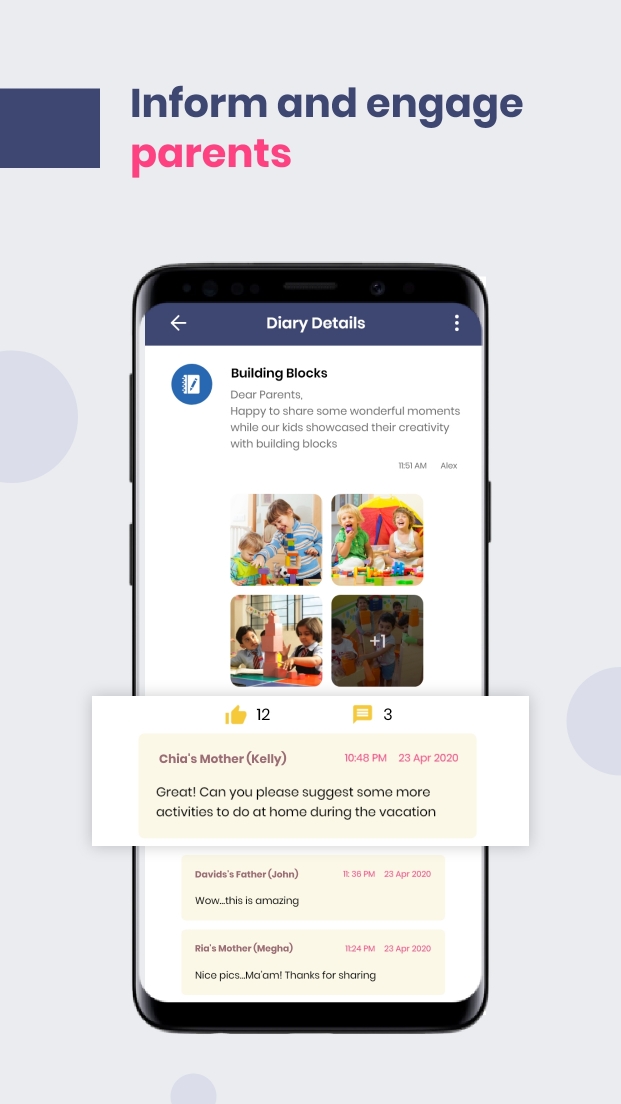The image appears to be a screenshot from a website with a predominantly light bluish-gray background. Along the left side, approximately one inch from the top, there is a small blue tab that extends over by an inch, moves downward by an inch, and then exits to the left. On this tab, the text "inform and engage" is written in dark blue, while "parents" is displayed in pink beneath it.

From the blue tab, about two inches down, a very light blue semi-circle intrudes from the left edge of the image. Similarly, another light blue semi-circle emerges from the right edge, situated approximately two inches from the bottom.

Centered within the image is a depiction of a smartphone, whose top edge is about two inches above the bottom of the image. The phone features a black border that encompasses its top, sides, and bottom. At the top of the phone's screen, a blue bar with a white arrow on the right edge is visible. The text "Dietary Details" appears in white on the left side of the blue bar, accompanied by a vertical trio of dots on the right.

The majority of the phone's screen is white. Displayed at its top left corner is a blue circle containing an icon of a white notepad and a blue pencil. To the right of this icon is the bolded text "Building Blocks." 

Beneath "Building Blocks," there is a message that reads: "Dear Parents, happy to share some wonderful moments while our kids showcase their creativity with building blocks," formatted across four lines. To the lower right of this message, the timestamp "11:51 AM" and the sender's name, "Alex," are shown.

Below the message, four images depicting kids are arranged, followed by a rectangular tab that stretches horizontally beyond the phone's boundaries. This tab indicates "12 likes" and "3 comments." Further information is written underneath this section, accompanied by two additional tabs that are still within the phone's display and have not been extended outward.